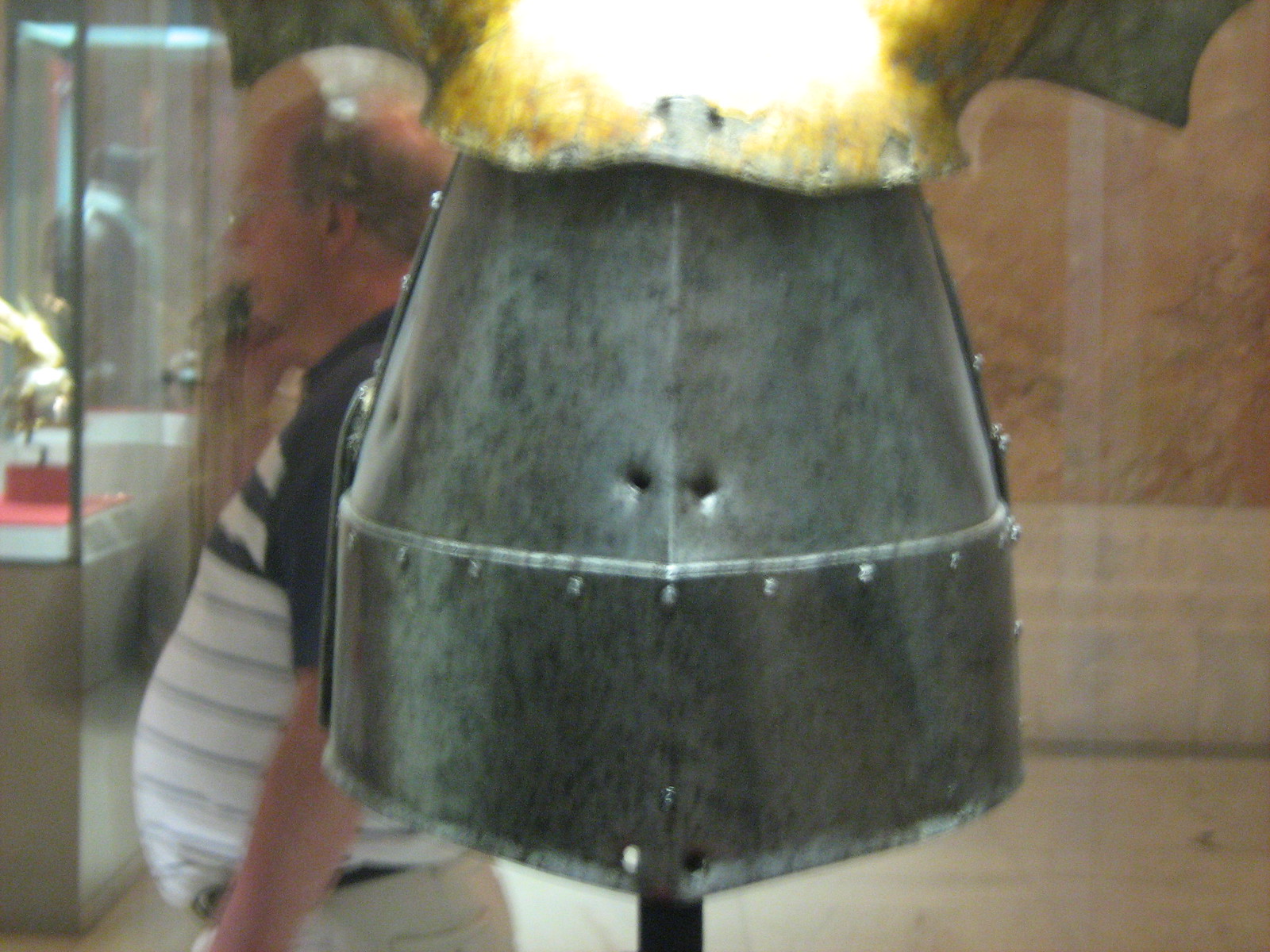In this grainy image, a reinforced metal pot or kettle, prominently positioned in the foreground, captures immediate attention. Flames appear to be erupting from its top, adding a dynamic element to the scene. The pot's sturdy steel is bolstered by bolts along its sides and base, forming a conical shape. A stick props up the pot, suggesting it might be part of a traditional cooking setup.

In the background stands an elderly gentleman, dressed in a short-sleeve collared shirt. The shirt is notably divided into two sections: a dark blue upper portion and a white lower section adorned with stripes, while the sleeves remain a solid blue. The man wears glasses and has a receding hairline, indicating some baldness at the front. His outfit is completed with beige pants and a dark-colored belt. Behind him, a glass display case adds an additional layer of depth to the scene.